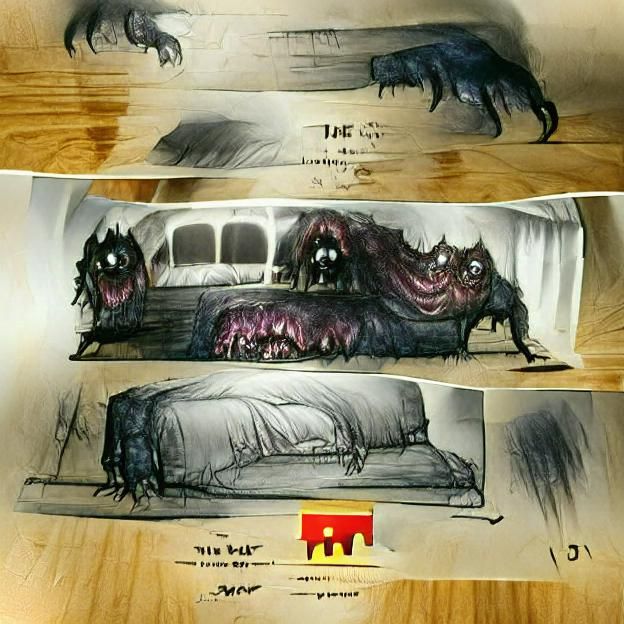The three sequential images depict a detailed and eerie narrative set on a wooden backdrop. The top image illustrates a tapestry featuring grotesque ghouls with purple faces, black bat wings, and sharp talons emerging from a white void. Accompanied by unreadable text, the monsters appear to be crawling out from their confinement. The middle image portrays a group of these nightmarish creatures, blending into a frightening mass of black fur and red flesh, seemingly seated on a couch within a white tent that has black windows. In the final image, the monsters have vanished entirely, leaving behind a dirty white fabric covering, adorned with some black marks resembling unreadable text and a distinct red and yellow square design at the bottom. The narrative is intriguingly mysterious, raising questions about the creatures' disappearance and their ultimate fate.